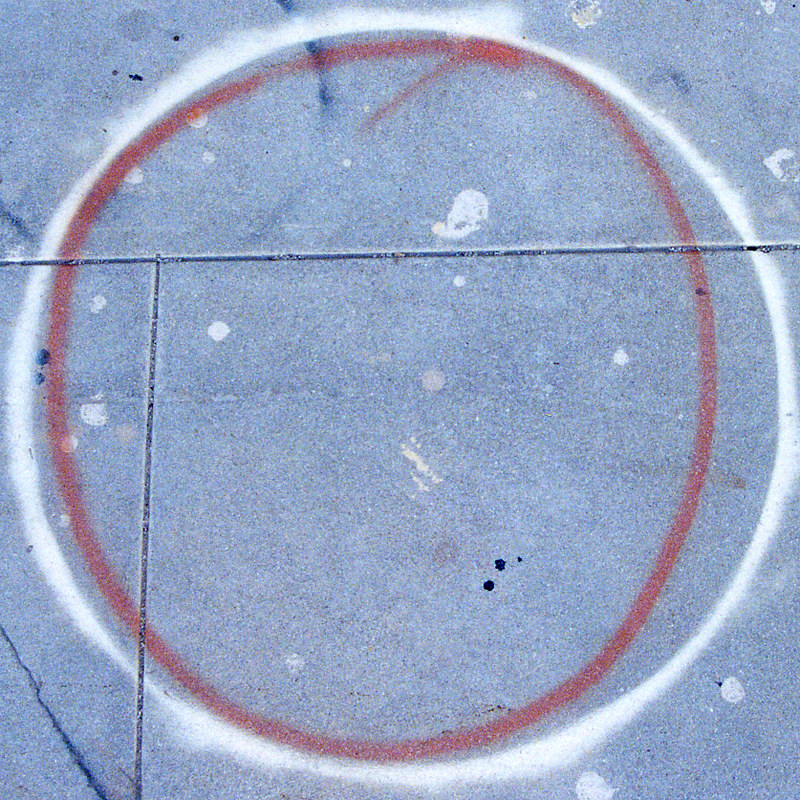This photographic image captures a section of a gray pavement or concrete wall outside a building. The surface, composed of gray concrete blocks with visible cracks and grout lines, appears weathered and textured. The main feature of the image is vibrant graffiti consisting of concentric circles. The outer circle is white, and within it is a smaller red circle. Scattered within the red circle are several white splotches, mostly circular, but one irregular in shape at the top. Additionally, there are three distinct black dots inside the circles. The area outside the white circle features more splotches, predominantly in the bottom right-hand corner and a few in the top right-hand corner. A striking black mark, partially cutting into the white and red circles, is noticed at the top with a red line adjacent to it. A partial, darker navy blue ring is observed in the left-hand corner, adding to the array of colors and textures that make up this intriguing graffiti scene on the gray, lined concrete surface.